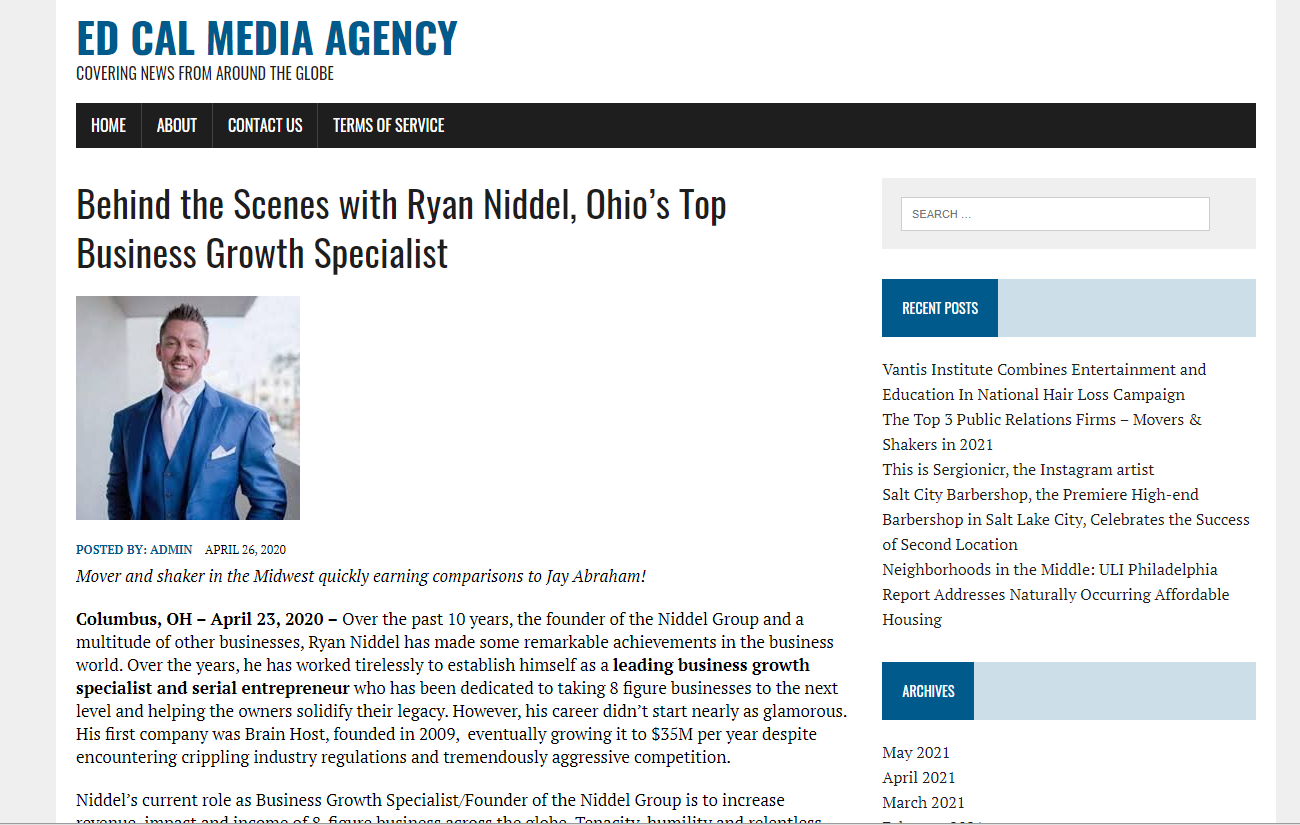The image features a webpage from EdCalMediaAgency, prominently displayed in the top left corner with large blue font. Beneath the logo, the tagline "Covering news from around the globe" is visible. A black banner spans the width of the page below, containing navigation links: Home, About, Contact Us, and Terms of Service.

The main story headline, "Behind the Scenes with Ryan Nadell, Hawaii's Top Business Growth Specialist," dominates the central portion of the page, accompanied by a photograph of Ryan Nadell. The article is written by Admin and was posted on April 26th, 2020. The text body includes several bolded phrases, notably "Columbus OH, April 23rd, 2020," "Leading Business Growth Specialist," and "Serial Entrepreneur."

On the right-hand side, a small grey panel towards the top contains a site search feature. Directly below this, a banner, featuring a dark blue section on the left and a light blue section on the right, is labeled "Recent Posts." Following the recent posts text, another banner resembling the first one but listing "Archives" appears further down the page.